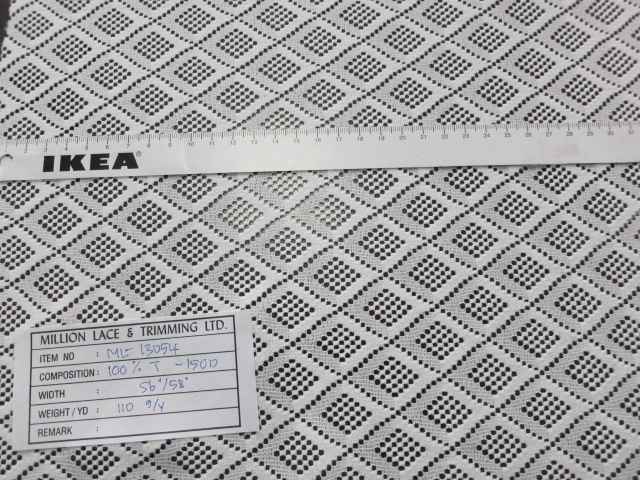The image features a detailed, white lace fabric characterized by a pattern of diamond shapes, each containing a grid of smaller lacy circles. The diamonds appear half light gray and half white on the right side, creating a textured and intricate design. The fabric is displayed on a black background, making the holes in the lace stand out prominently. A piece of paper in the lower left corner bears detailed information: it reads "Million Lace and Trim LTD, Item number ML13054, Composition 100% T-150D, Width 56-58 inches, Weight 110 grams per yard," with a remark field that is blank. Additionally, an IKEA yardstick is placed on the fabric, with the bold black IKEA logo clearly visible on the left side.